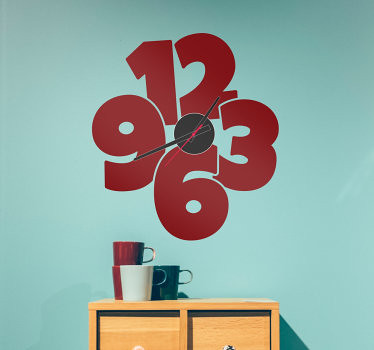This digital artwork features a realistic depiction of a light wood-colored piece of furniture with two square drawers at the bottom, each with visible top handles. The left handle is completely white, while the right handle is white with a black section. On top of the furniture are four coffee cups arranged in a slightly overlapping manner. To the left, there are two red coffee cups stacked one inside the other, each with a gold handle pointing to the right. In front of these is a white coffee cup with a green handle pointing to the right. Behind the white cup is a green coffee cup with a silver handle, also pointing to the right.

The background of the image is a greenish-blue or teal color. On this background, there is a stylized clock with large deep red numerals: 12 at the top, 3 to the right, 6 at the bottom, and 9 to the left. These numbers are arranged in a clockwise direction around a central black circle. Inside this black circle are traditional clock hands: two long black hands and a thin red minute hand, indicating the time. The entire composition is unified by the contrasting colors and structured arrangement of the elements.